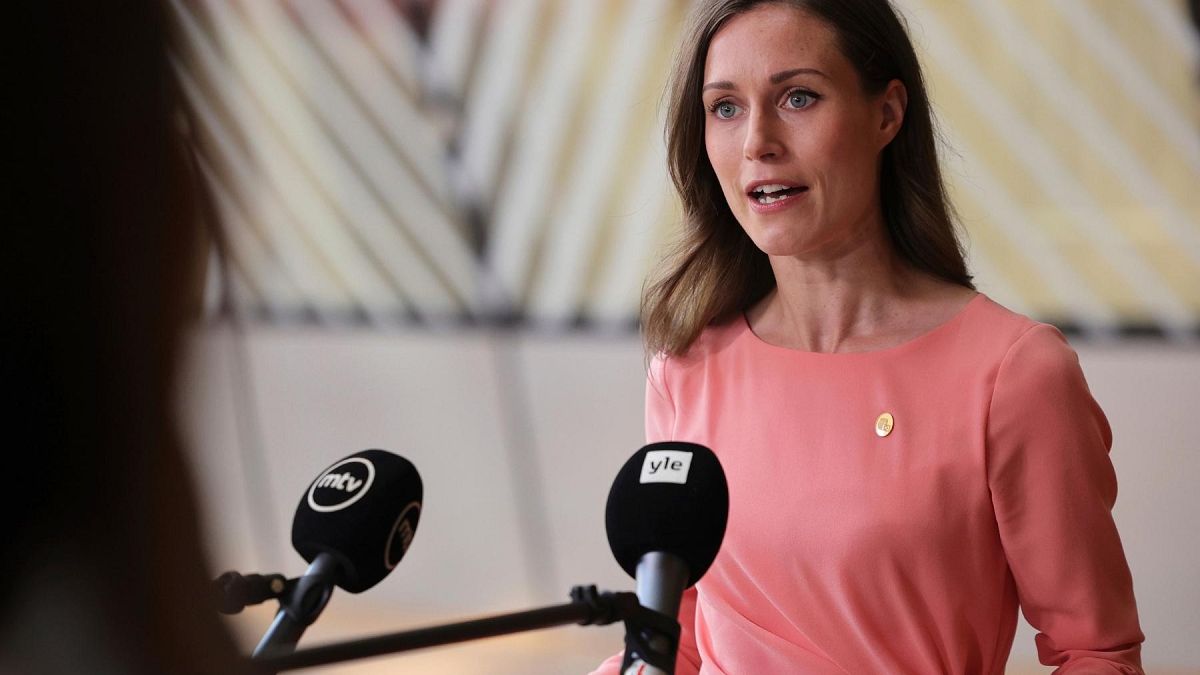The image depicts a woman, likely at a press conference, speaking into two microphones positioned in front of her. The microphones have large black foam tips; the one on the left is labeled with a white circle reading "MTV," and the one on the right has a white square displaying "YLE." The woman has long, straight brown hair, parted in the middle, with blue eyes and is wearing pink lipstick. She is dressed in a long-sleeve, coral or salmon-colored shirt, adorned with a small, circular gold pin on her left chest. Her mouth is open, suggesting she is in the middle of speaking or making a statement. 

The background features a blurry wall with alternating diagonal lines of yellow and white stripes at the top, transitioning to a cream color with additional golden yellow stripes further left. A shadowy figure with strands of hair appears on the left edge of the image, though it’s not entirely clear if it is another person. The visual elements provide a dynamic and somewhat busy scene, focusing on the woman as she addresses the audience.